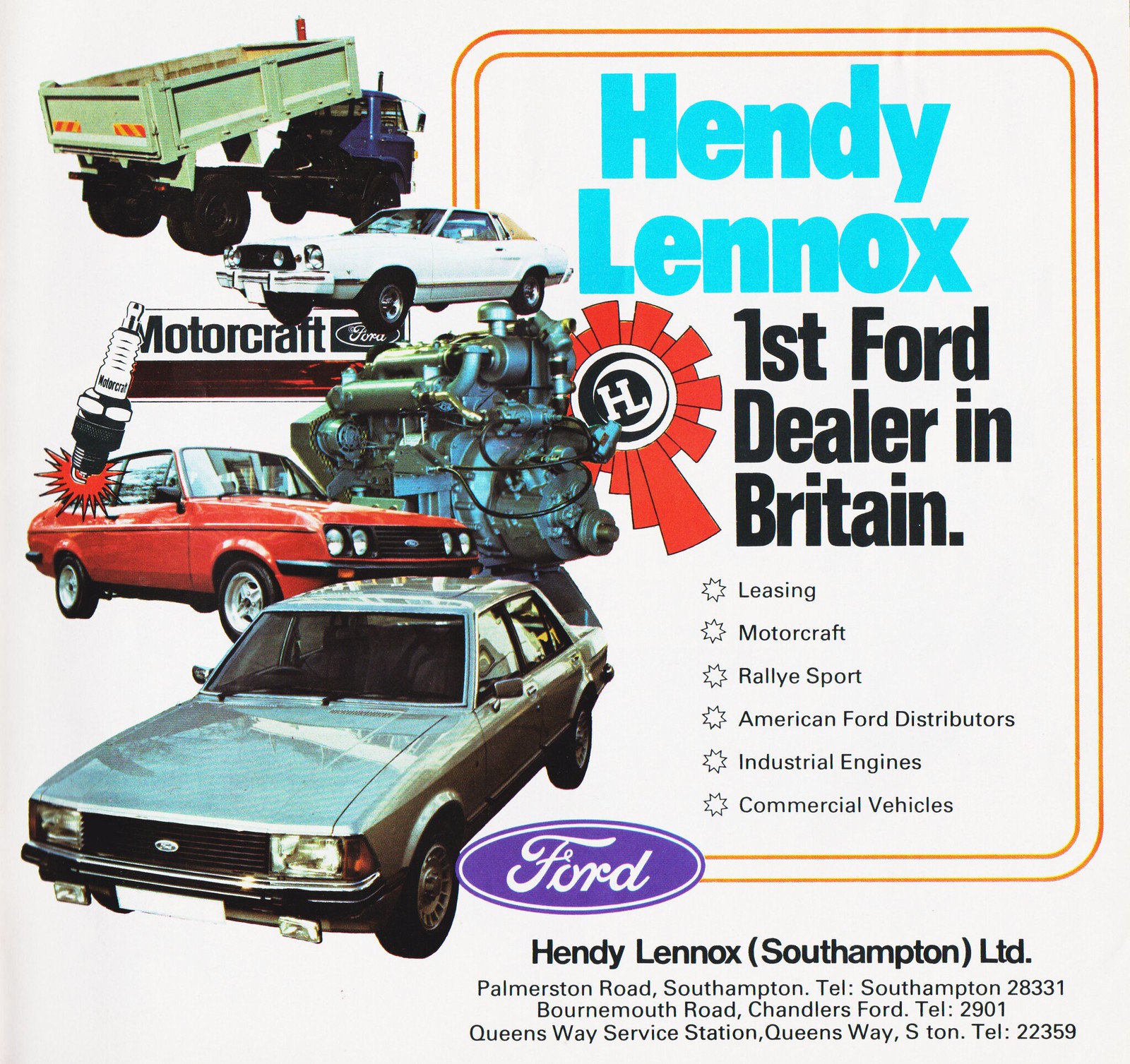This is a digital image of a vintage advertisement from an old magazine for Hendy Lennox, the first Ford dealer in Britain. On the left side, the poster features colorful pictures of various vehicles and automotive components. At the top left, there is an image of a dump truck followed by a series of smaller photographs, including a white Ford Mustang, a spark plug, an engine, a red coupe, and a greenish gray car. These images are displayed over a Motorcraft Ford logo. 

The right side of the poster has text with a heading in blue that reads "Hendy Lennox," followed by a subheading in black text: "First Ford Dealer in Britain." The text below this heading is organized into bullet points listing services and offerings: "Leasing, Motorcraft, Rally Sport, American Ford Distributors, Industrial Engine, Commercial Vehicle." This section of text is framed by two orange borders. Beneath the bullet points is the classic blue oval Ford logo.

At the bottom of the text section, the contact information for Hendy Lennox, Southampton Limited is provided, including their address and phone number. This entire advertisement is set against a light gray background.